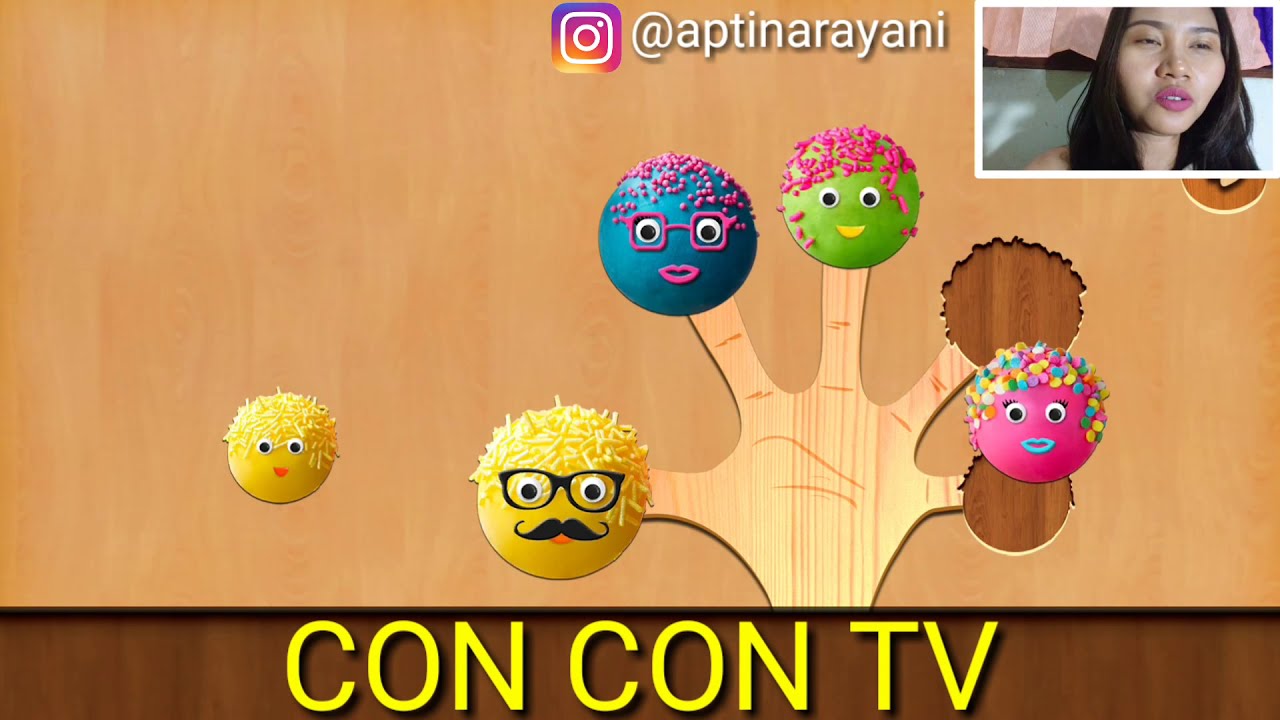The image entitled "ConConTV" features a central cartoon drawing on a light brown wooden background, resembling a tree with five branches. Each branch displays a round, smiley cartoon face like a colored sphere, each with unique features: 

- The thumb has a yellow circle with googly eyes, glasses, a mustache, and sprinkles on its head.
- The index finger has a blue circle with pink glasses and lips.
- The middle finger has a green circle with yellow lips and no glasses.
- The ring finger has a pink circle with blue lips and multicolored hair.

Towards the bottom, a brown bar spans from left to right displaying the text "ConConTV" in yellow letters. In the upper right corner of the image, there is a small photograph of an actual woman with chubby cheeks, black shoulder-length hair, and pink pouting lips against a light blue background. Above her photo, an Instagram icon appears next to the handle "@Appianaryani".